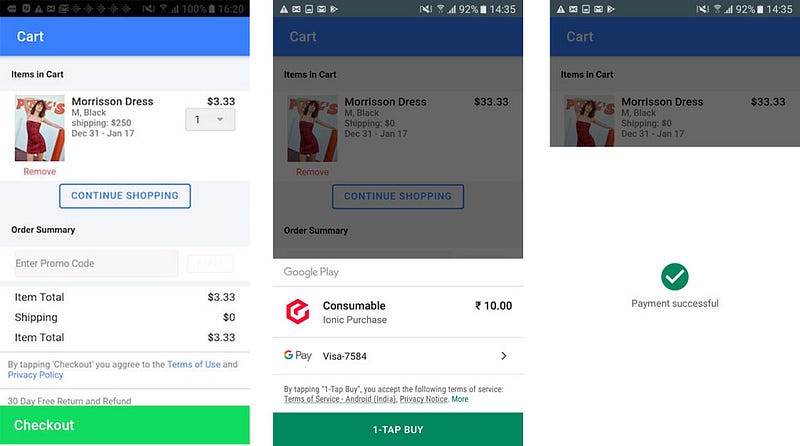The image shows three consecutive screenshots of an individual shopping on their cell phone, providing a detailed journey from cart viewing to purchase completion.

In the first screenshot, the top of the cell phone screen displays various indicators, including the battery life, signal strength, Wi-Fi connection, and the current time. Below this, a black bar contains minimal information, while a prominent blue bar with white text denotes the section title "Cart." Under this, the details of items added to the cart are visible. The main item listed is a "Morrison Dress" in size medium, black, priced at $3.33. Shipping costs are noted as $2.50, with an estimated arrival window from December 31st to January 17th. The interface provides options to remove the item, continue shopping, and also displays the order summary. There is an option to enter a promo code, and the total cost of the item, shipping fee, and final total are reiterated.

The second screenshot mirrors much of the information from the first but also includes additional payment method details. Here, it specifies payment via Google Pay, with an item labeled "Consumable Ionic Purchase" costing $10. The payment method is confirmed as a Visa card ending in 7584. The system informs the user that by tapping "One Tap Buy," they accept the terms of service. The "One Tap Buy" button is prominently displayed for user action.

In the third and final screenshot, the purchase confirmation is highlighted. The previously mentioned items and their details remain, now supplemented with a "Payment Successful" message. This confirmation is set against a green background with a white checkmark, clearly indicating that the transaction has been completed successfully.

The screenshots collectively provide a comprehensive look at the online shopping process, starting with item review, moving through payment details, and culminating in purchase confirmation.